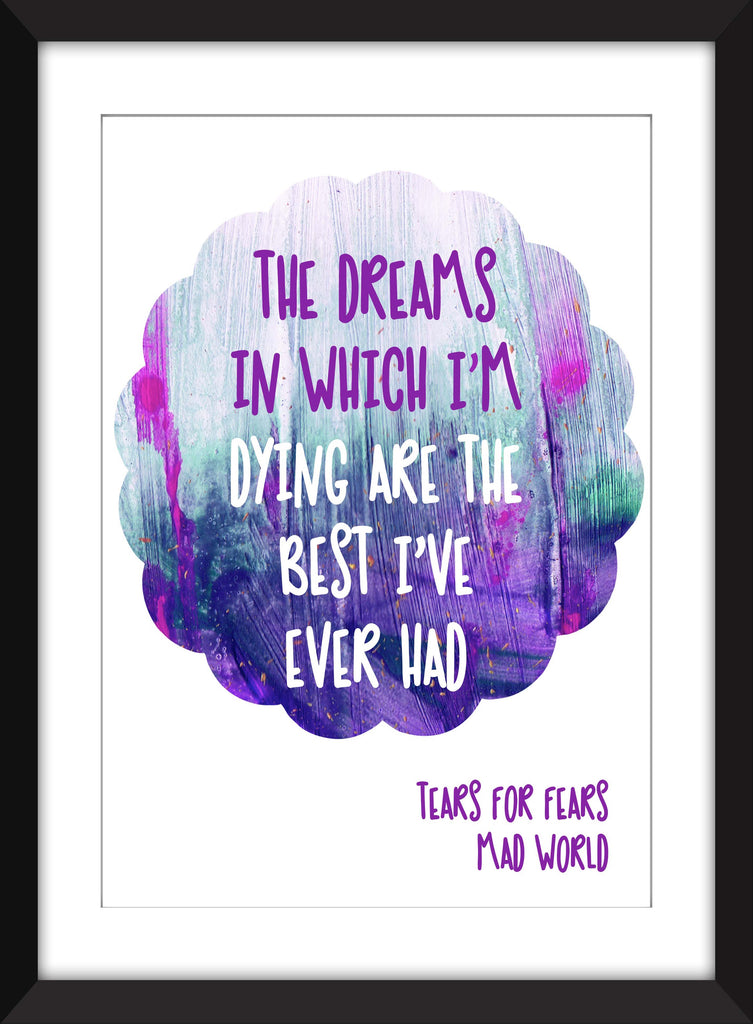This image showcases a vertically oriented art print encased in a black frame with a white mat. The centerpiece of the print is a purple and blue ombre circle with scalloped edges, creating a whimsical cloud-like shape. Inside this shape, in a handwritten, whimsical font, it reads, "the dreams in which I'm dying are the best I've ever had," with "the dreams in which I'm" rendered in purple text and "dying are the best I've ever had" in white. Beneath this ombre circle, against the white background of the poster, the text "tears for fears mad world" is inscribed in purple on the bottom right corner. The print, featuring tones of purple, magenta, and gray, appears to be a product image, perhaps intended for sale on a website, set against a simple white background. The text on the poster refers to lyrics from the famous song "Mad World" by Tears for Fears.